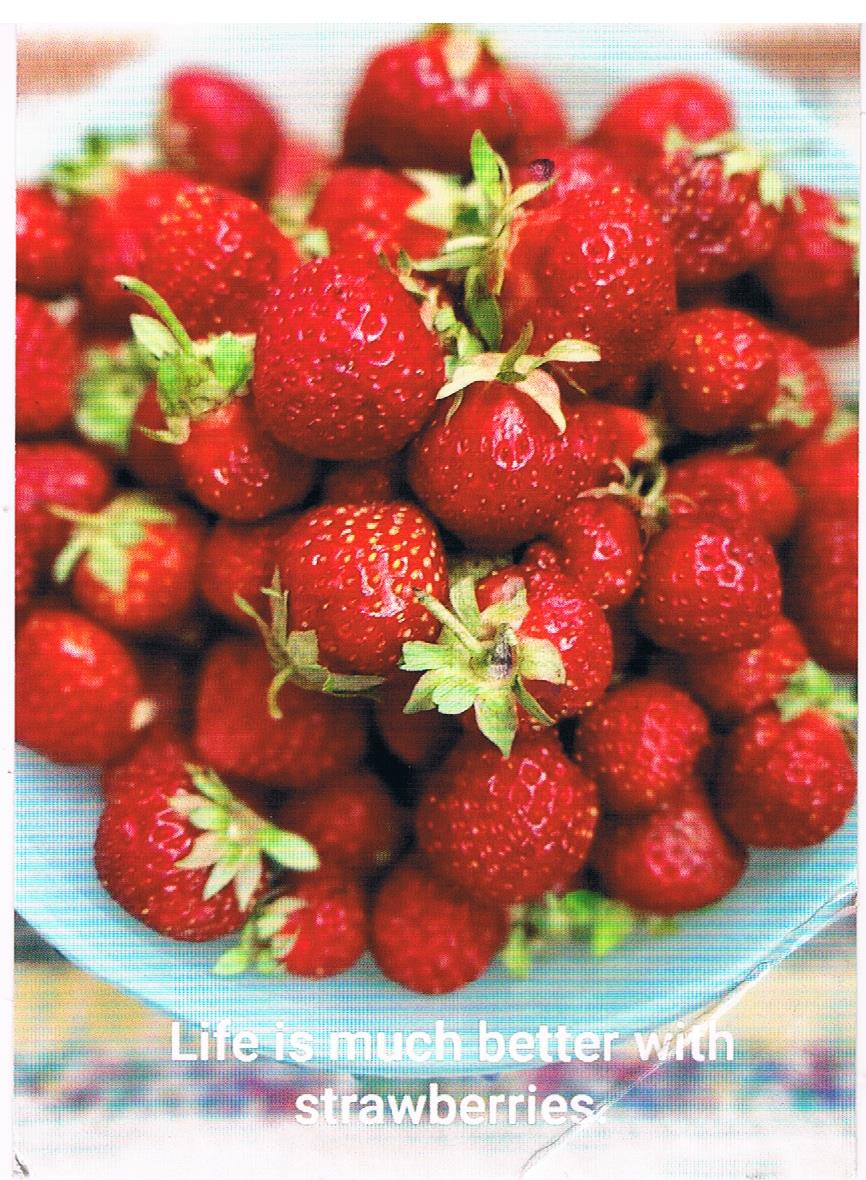The image captures a bowl brimming with strawberries, each still bearing its green stems, suggesting they might not have been completely cleaned. The strawberries vary in condition; some appear fresh, while others show signs of bruising or age. The container holding the strawberries is a light blue bowl, prominently centered in the image and occupying most of the frame. The white text at the bottom of the image reads, "Life is much better with strawberries." The background is slightly blurred, revealing hints of yellow, purple, and green colors, suggesting a tablecloth with floral patterns. The overall setting suggests an indoor table where the photo was taken, enhancing the fresh and homely feel of the scene.